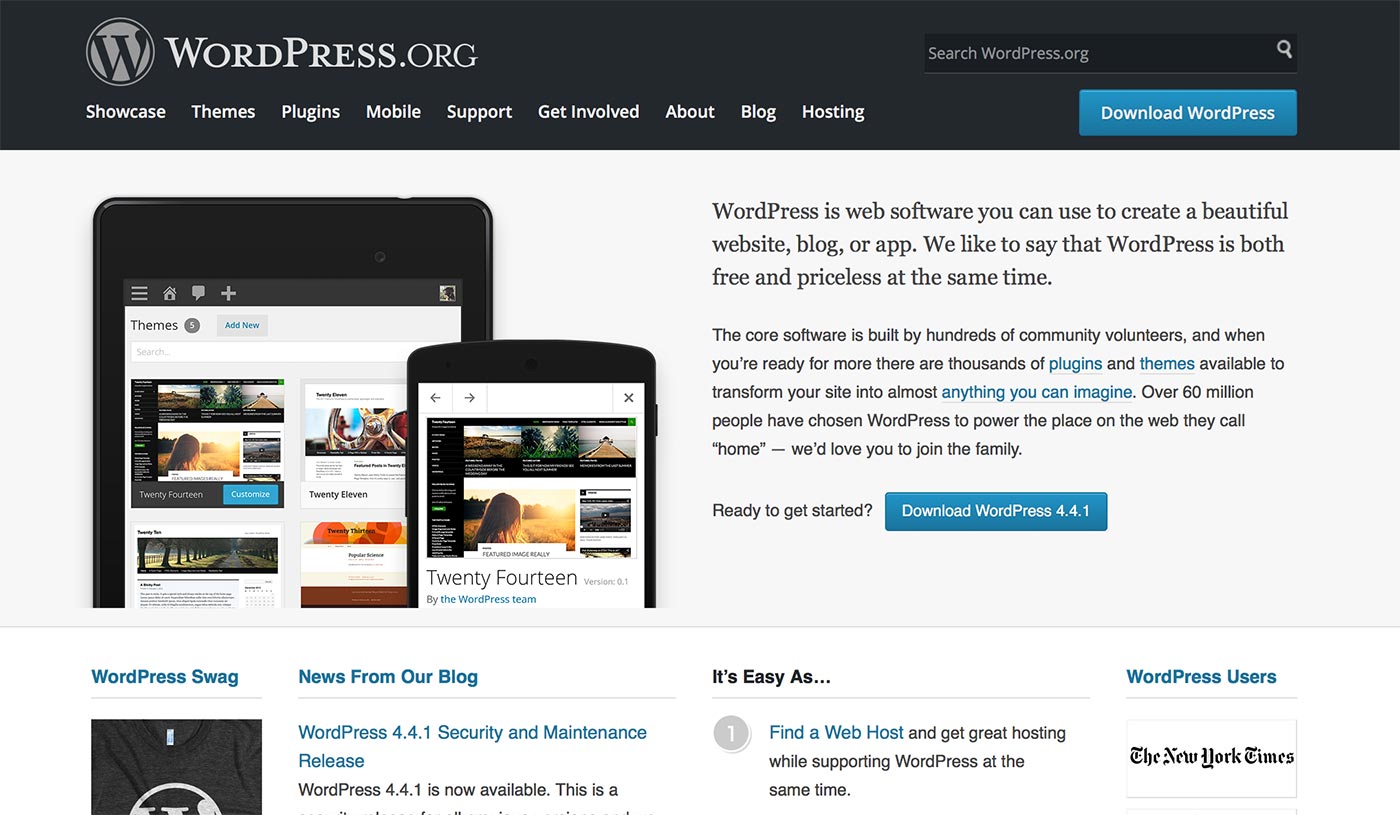The image depicts a detailed view of the WordPress.org website, as seen on a laptop screen. At the top of the page, a black banner prominently displays the WordPress logo accompanied by the text "WordPress.org." Below this banner is a navigation menu with several links: Showcase, Themes, Plugins, Mobile Support, Get Involved, About, Blog, and Hosting. 

On the right side of the menu bar, there is a rectangular button labeled "Download WordPress." Directly above this button is a search bar featuring a magnifying glass icon on the right. 

The main content area of the page shows two images of devices on the left—one appears to be a Kindle, and the other is a different-sized Kindle-like device. To the right of these images, the headline "WordPress" is followed by a paragraph explaining that the core software is built by hundreds of community volunteers. It highlights that thousands of plugins and themes are available for users to customize their sites.

Further down, there is a prominent button labeled "Download WordPress 4.4.1." The bottom section of the page breaks into segments featuring various articles and links, including "WordPress Swag," "News from our blog," "It's Easy As," and "WordPress Users."